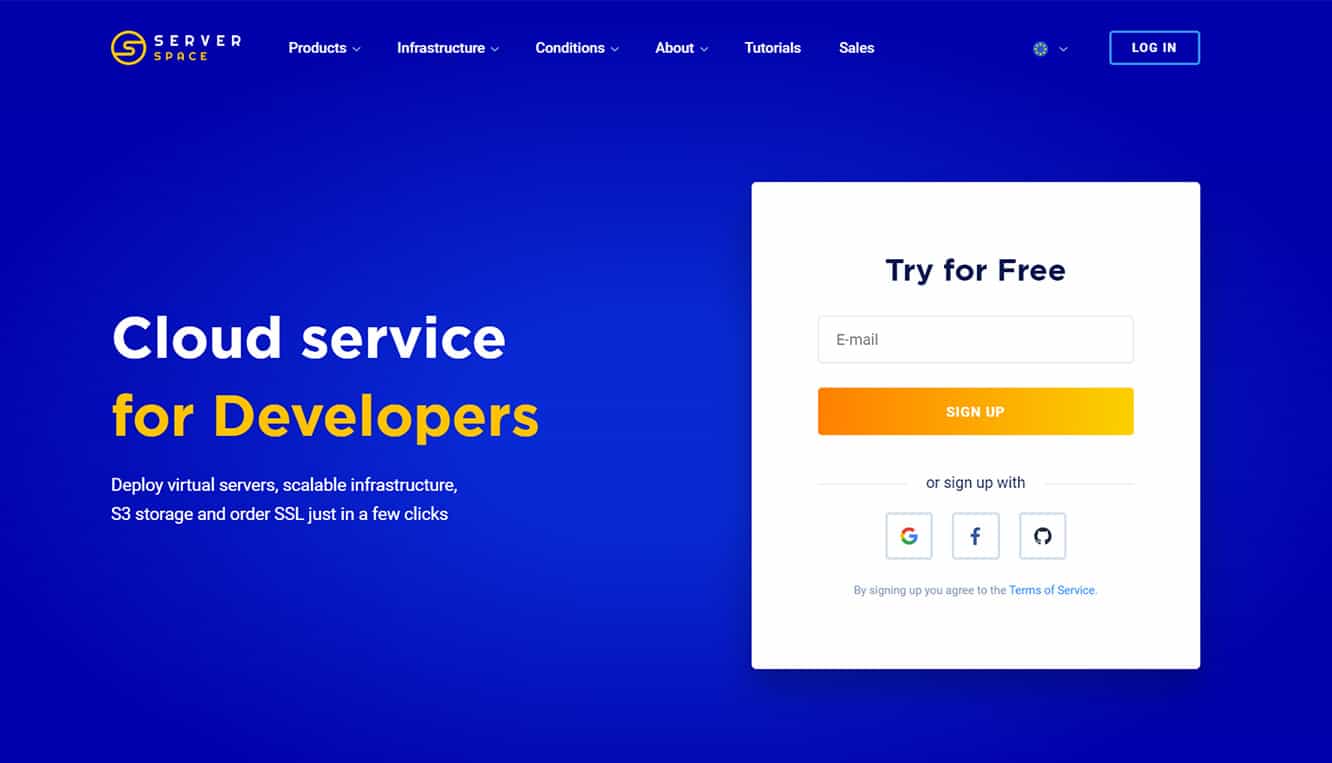This is a detailed caption for the given image description:

---

A screenshot captured from a desktop PC monitor or tablet depicts a webpage with a medium royal blue background devoid of any title or taskbars. Dominating the top is a distinctive logo, featuring a yellow circle with an "S" inside, set against a blue background, suggesting the brand name "Server Space." The page header displays several navigation options in white text, including "Products," "Collections," "About," and other categories that are difficult to discern due to their small size. A "Log In" option is also prominently available.

In the main content area, bold white text reads "Cloud Service," with the supplementary tagline "For Developers" in yellow beneath it. To the left, there is a white rectangular box with the text "Try for Free" in black. Below this, users can enter their email address into an input field, accompanied by an orange rectangular button with "Sign Up" in white text. Additional sign-up options include icons for Google and Facebook, as well as another unidentified symbol.

Further down, promotional text elaborates on the features of the service, stating, "Deploy virtual servers, scalable infrastructures, S3 storage, and code SSL — all in just a few clicks."

---

This enhanced caption provides clear and detailed context, ensuring the reader can easily visualize the screenshot.